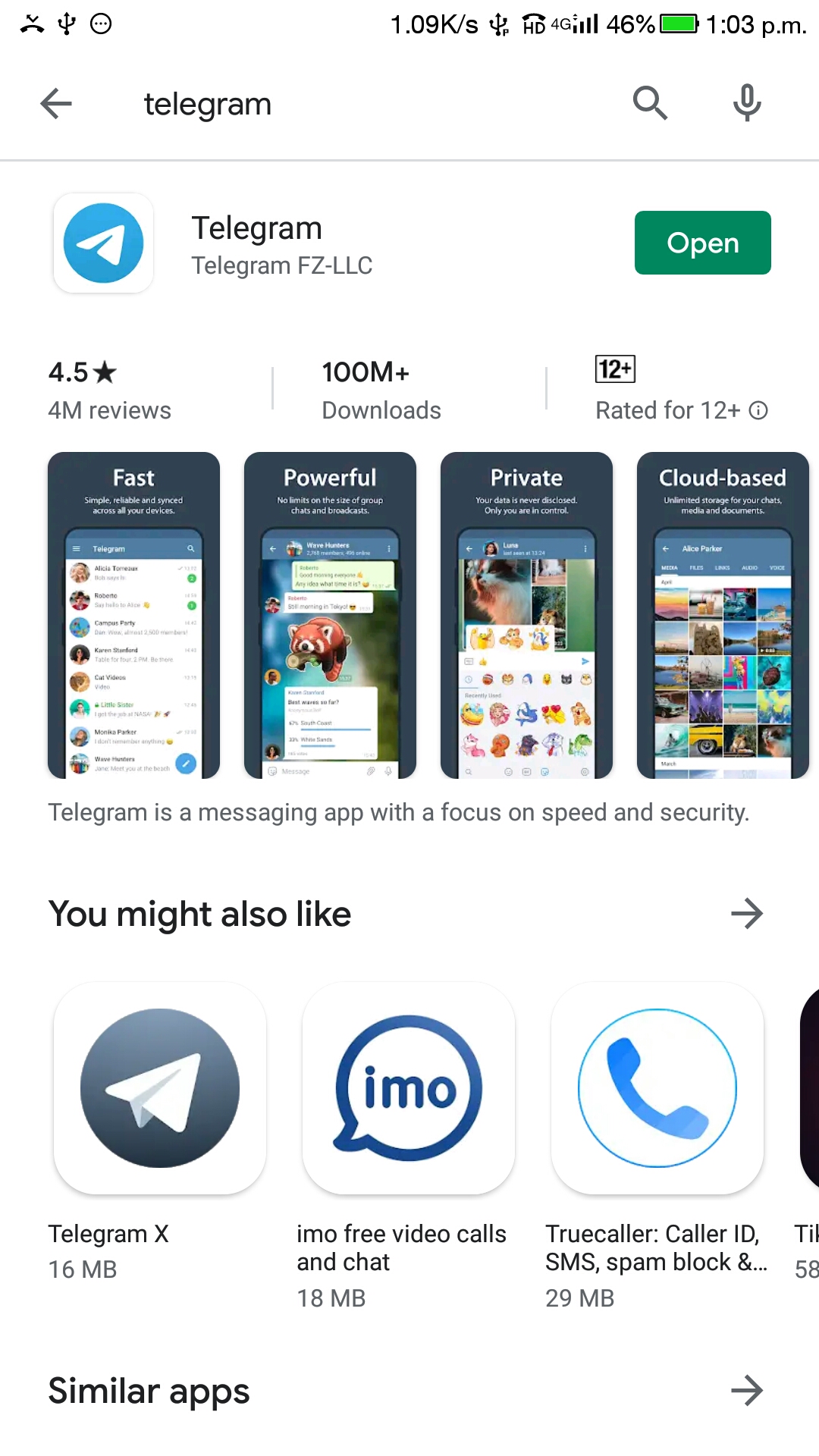The image depicts a screenshot of the Telegram app's information page from a mobile device. The screenshot is taken at 1:03 PM, with the phone's battery at 46% and showing a connectivity status. The top of the screen displays "Telegram" with the label "FZ LLC" beneath it. Below this, a green "Open" button is highlighted, indicating the app is already installed or ready to be opened.

The screen features a white background with several review highlights indicating the app’s strengths: "Fast," "Powerful," "Private," and "Cloud-Based." It is also noted that Telegram has garnered over 4 million reviews with an average rating of 4.5 stars, has been downloaded more than 100 million times, and is rated suitable for ages 12 and up. The description beneath these highlights emphasizes Telegram's focus on speed and security.

At the bottom of the image, there are suggestions for similar apps to Telegram, including "Telegram X," "IMO free video calls and chat," and "Truecaller," the latter depicted with an icon showing a phone inside a circle and noted for its Caller ID and SMS spam block functionalities. The fourth recommended app is partially cut off, only showing a black section along with the phrase "similar apps" and an arrow pointing to the right.